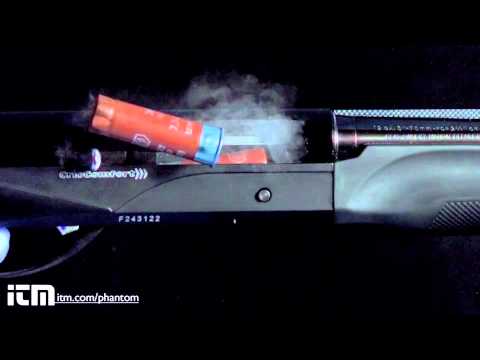The image is an up-close shot of a dark-colored car dashboard. Prominently featured on the right-hand side is a speaker, and above the dashboard is a red cylindrical object resembling a bullet casing with a metallic blue base. The cylinder appears to be falling towards the left, with its bottom already touching the dash while the top is still slightly suspended, surrounded by a puff of smoke. The dashboard also includes visible signage, displaying "F243122" and a label in white reading "ICN" along with the website "itm.com/phantom" in the bottom left corner.